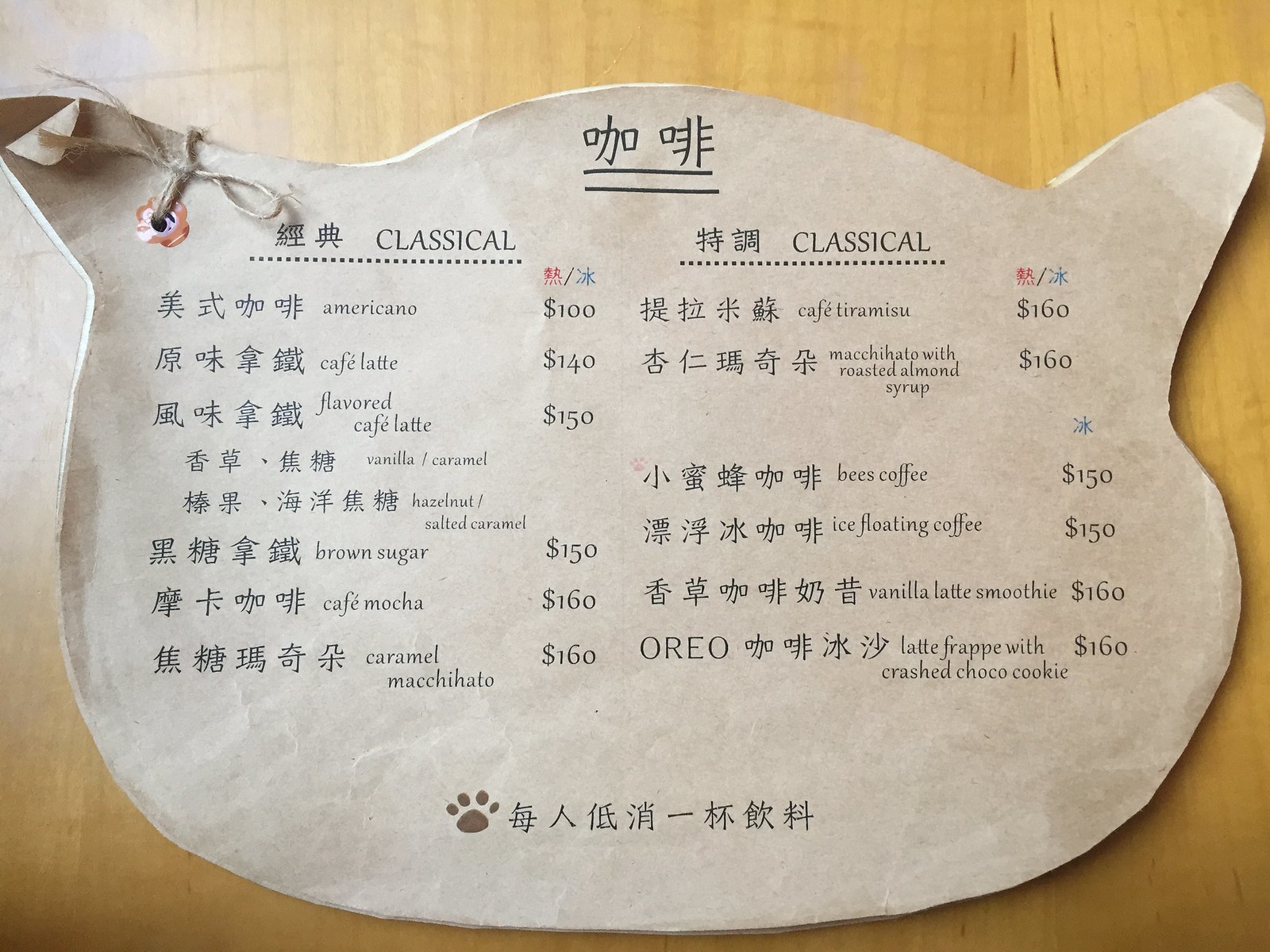This photograph captures a uniquely designed menu, predominantly featuring Chinese text with some English translations. The menu is printed on thick, off-white, manila paper with a distinctive eye hole reinforced with a protector and threaded with twine. The menu's top edge is artistically shaped to resemble a cat’s face, complete with ears.

Under the written descriptions, the drink offerings are meticulously listed, covering a range of coffee options and their prices:
- Americano: $1.00
- Cafe Latte: $1.40
- Flavored Cafe Latte (options include vanilla caramel, hazelnut, salted caramel, and brown sugar): $1.50
- Cafe Mocha: $1.60
- Caramel Macchiato: $1.60
- Cafe Tiramisu: $1.60
- Macchiato with Roasted Almond Syrup: $1.60
- Coffee: $1.50
- Iced Floating Coffee: $1.50
- Vanilla Latte Smoothie: $1.60
- Latte Frappe with Crushed Cocoa Cookie: $1.60

At the bottom of the menu, there is a bear paw print and additional Chinese writing, presumably reiterating the drink descriptions or perhaps providing extra information.

This menu not only provides a list of delicious beverages but also exudes a sense of classical and charming aesthetics through its careful design and thoughtful details.